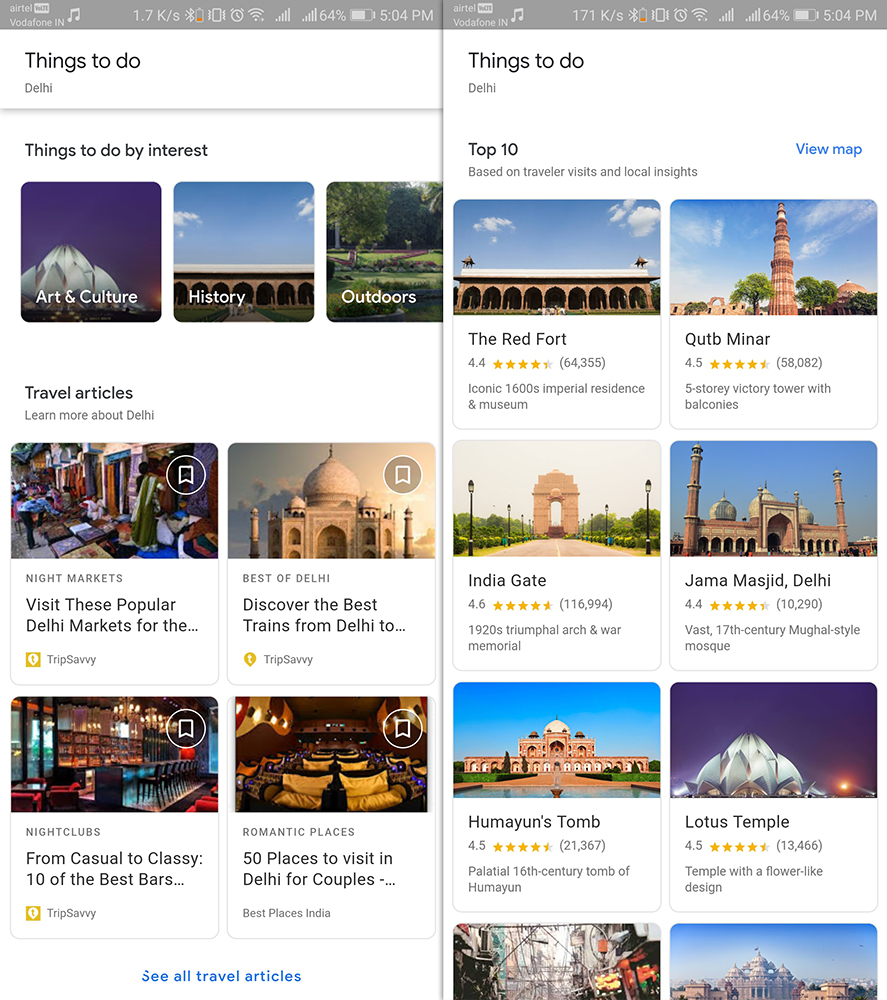**Detailed Caption:**

The image falls under the category "Websites" and showcases two smartphone screens displayed side by side. Both screens are running a music application. A detailed status bar is visible on each phone, showing that the devices are on vibrate mode, WiFi is enabled, and the battery level is at 64%. The current time shown is 5:04 PM.

The content on the screens pertains to activities and attractions in Delhi. The first screen features sections such as "Things to do in Delhi" and "Things to do by interest," with subcategories that include "Arts and Culture," "History," and "Outdoors." This screen also suggests travel articles like "Visit These Popular Delhi Markets," "Discover the Best Trains from Delhi," "From Casual to Classy: 10 of the Best Bars," and "50 Places to Visit in Delhi for Couples." Additionally, there is a prompt to "See All Travel Alerts" at the bottom.

The second screen highlights "Things to do" with a list of the "Top 10 Based on Traveler Visits and Local Insights." It also features an option to "View Map." Notable landmarks listed include the Red Fort, Qutub Minar, India Gate, Jama Masjid, Humayun's Tomb, and Lotus Temple.

**End Caption**